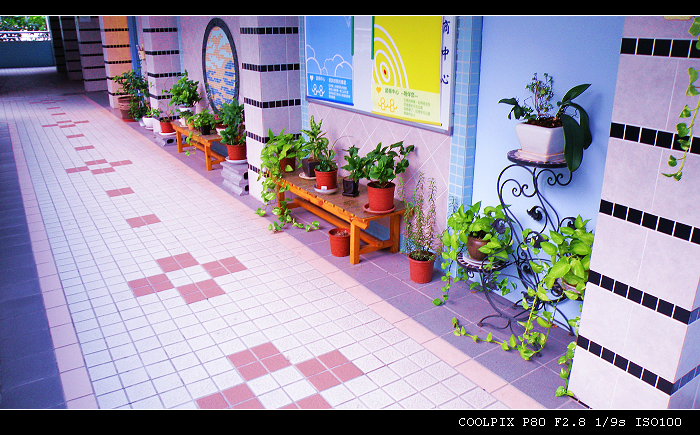The image is a vivid and colorful screenshot from a security camera, capturing a long, dynamic hallway with an intricate mosaic tile floor. The floor features a prominent thick white line running the entire length, surrounded by blue square outlines and intersected by red square tiles forming cross-like patterns. The walls add to the visual richness, adorned with a mosaic of a bonsai tree and sections painted in various shades, including pale blue, lavender with black trim, and orange trim. The hallway is furnished with orange wooden benches positioned against the walls, displaying an array of potted plants in red-orange plastic planters. Among the greenery are ivy vines and other green plants, contributing to the vibrant atmosphere. The overall scene suggests a communal space in a public building, school, or outdoor food court, characterized by its bold and colorful decor.